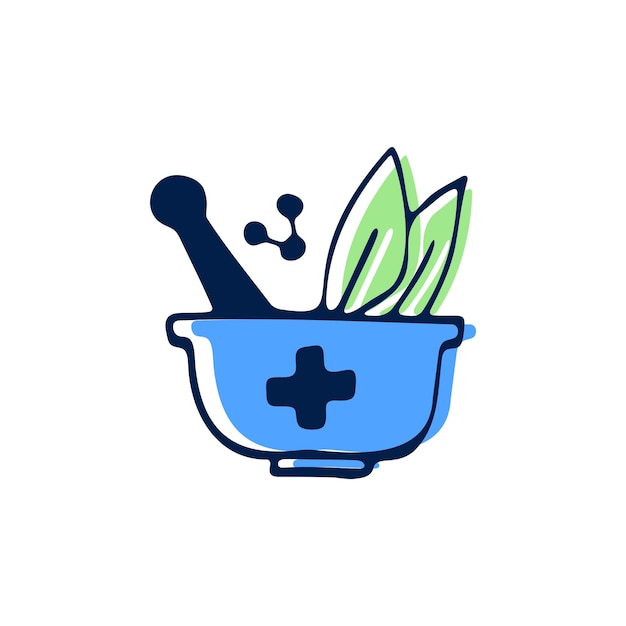The image is a digitally created illustration of a blue mortar and pestle set against a white background, enclosed by a dark blue border. The bowl, depicted in varying shades of blue, has a slightly misaligned, off-centered coloring with the darker blue primarily on the right side, leaving a white gap on the left. At the base, it features a rounded disc-like bottom with matching color discrepancies. A dark blue pestle, with a rounded top, extends from the bowl and leans towards the left. The front of the bowl showcases a dark blue cross symbol embedded within the light blue area.

Above the bowl, two green leaves, outlined and veined in a darker blue, protrude. The green within these leaves is similarly misaligned and offset to the right, creating a white space within the outlines on the left side. Positioned between the pestle and the leaves, three dark blue circles are connected by two lines forming a triangular pattern. The overall theme of the illustration suggests medicinal or health-related content, underscored by the plus sign and herbaceous elements.